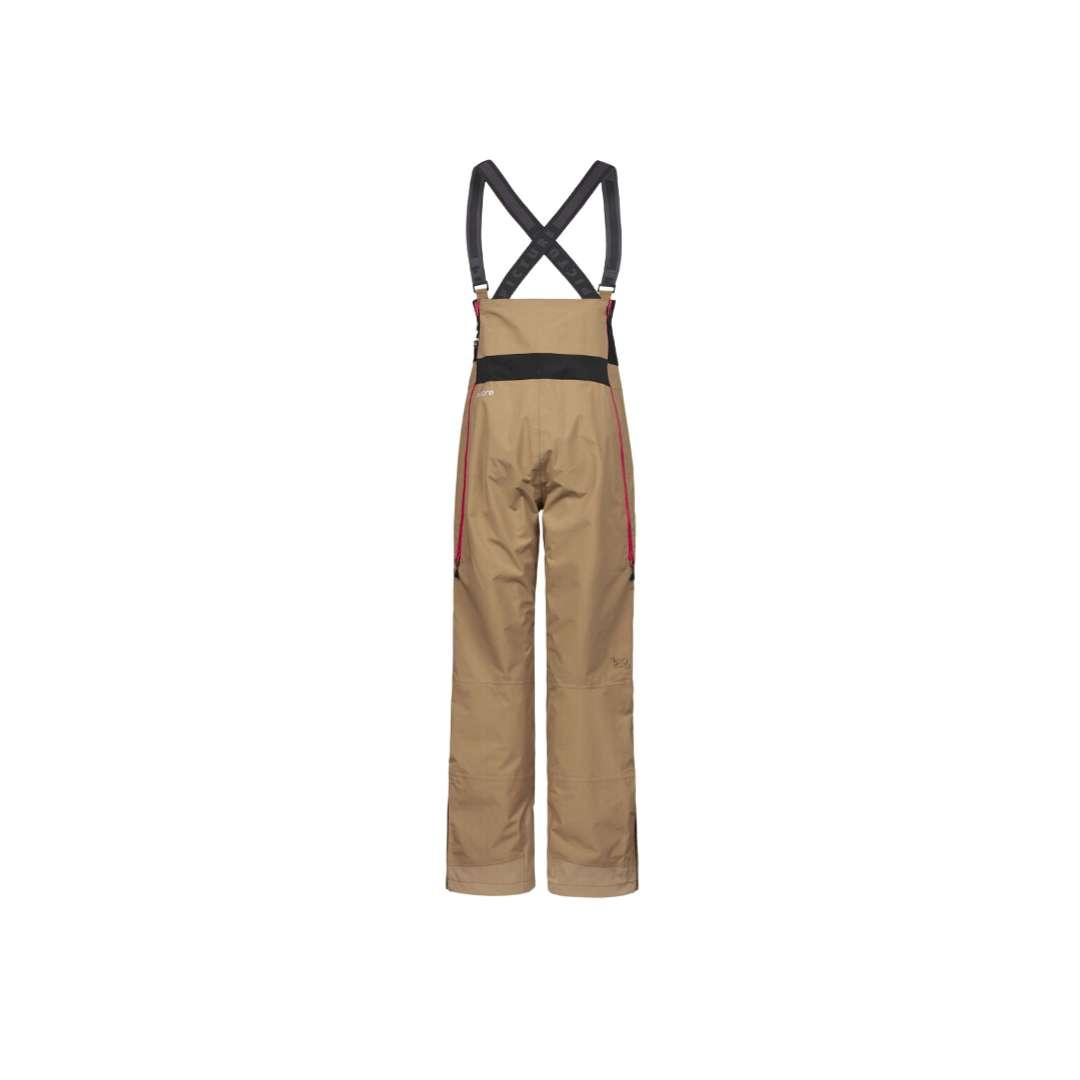This image depicts a pair of tan overalls set against a solid white background. The overalls are equipped with attachable black suspenders that are fastened with metal clips at the front. The trousers have a high waistline, likely extending up to the chest area. Running down both sides from the waist to the upper thigh are red zippers, adding a functional and decorative element to the garment. Additionally, the sides of the pants feature black sections and a black belt-like strap around the middle, providing contrast to the tan fabric. The overall design suggests they could be used for industrial purposes, outdoor activities, or possibly winter sports. The suspenders also feature a distinct pattern, enhancing their visual appeal. The arrangement of the overalls in the image gives the impression that they are being worn, although they are devoid of an occupant.